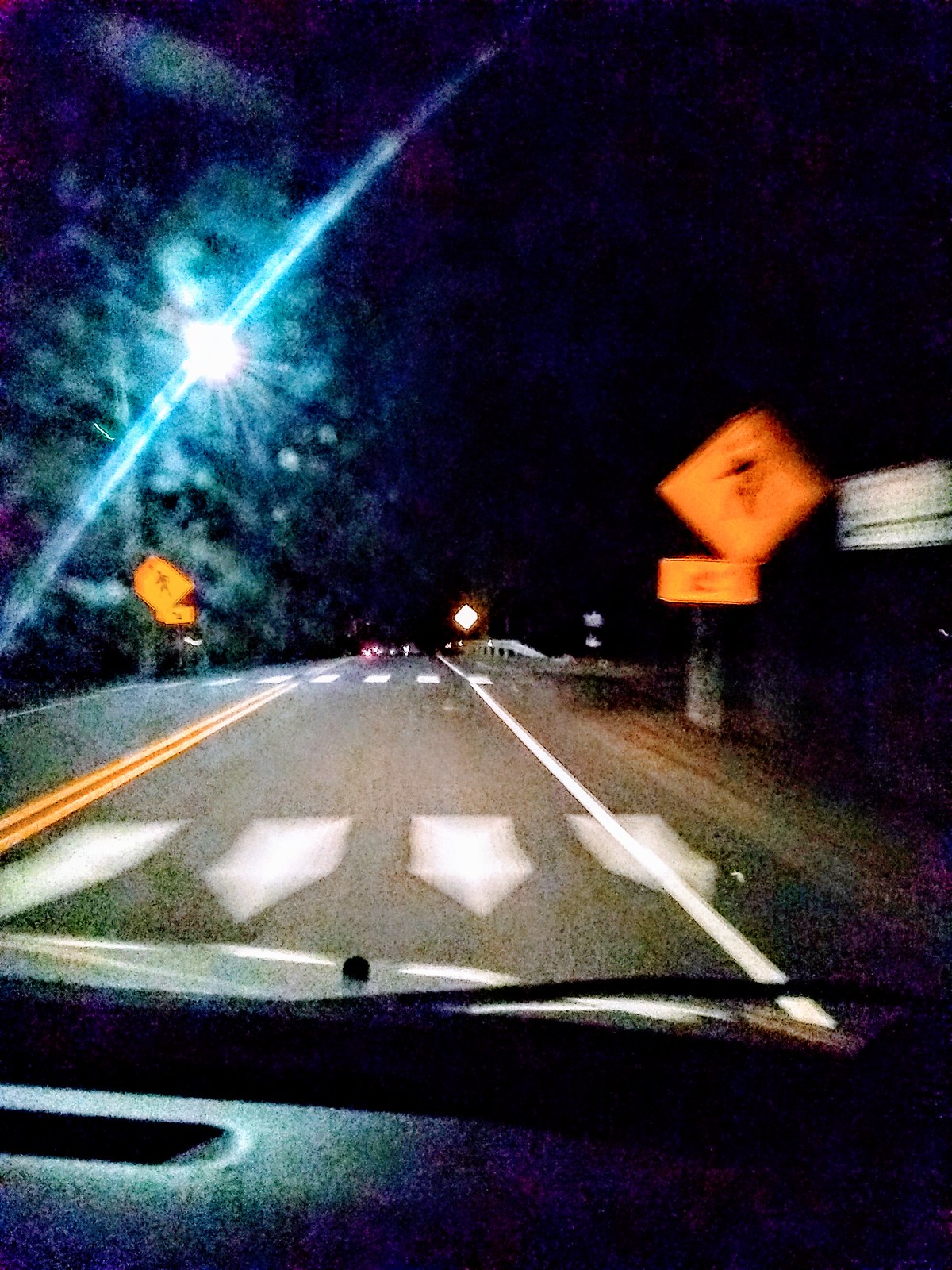A nighttime view captured through the windshield of a car driving in the right-hand lane of a highway. Near the right side, a yellow diamond-shaped traffic sign with an additional yellow rectangular sign beneath it is visible but too blurry to identify. On the left side of the road, a city light post casts beams of light that stretch diagonally across the scene, creating an atmospheric effect. White arrow markings on the pavement indicate directional flow, converging towards the car’s lane. Clearly defined road markings include a white line on the right side and double yellow lines separating the lanes. In the distant background, faint taillights of other vehicles illuminate the far reaches of the highway.